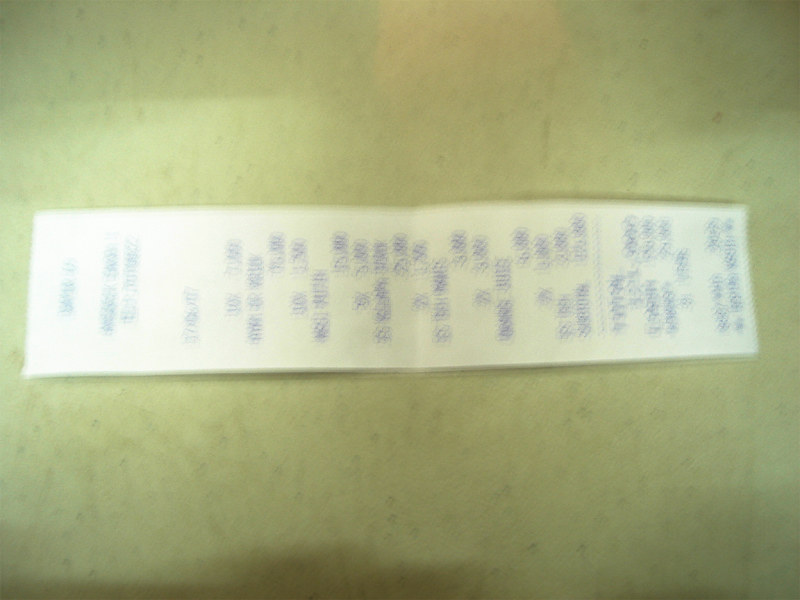The image showcases a highly zoomed-in shot of a light green surface, speckled with greyish-brown grains. Resting atop this surface is a long, rectangular receipt, folded in the middle. The paper appears white with navy blue and black writing. Positioned sideways, the top of the receipt faces the right-hand side of the picture, and there's a noticeable light glare, especially on the top-left section of the receipt. The text is oriented from top to bottom but arranged horizontally across the receipt. Despite attempts to discern the details, the writing remains blurry and partially obscured by the glare, making it difficult to read the exact items or numbers listed. There are also dotted lines horizontally crossing the top portion of the receipt, suggesting itemization and a thank-you note at the bottom.